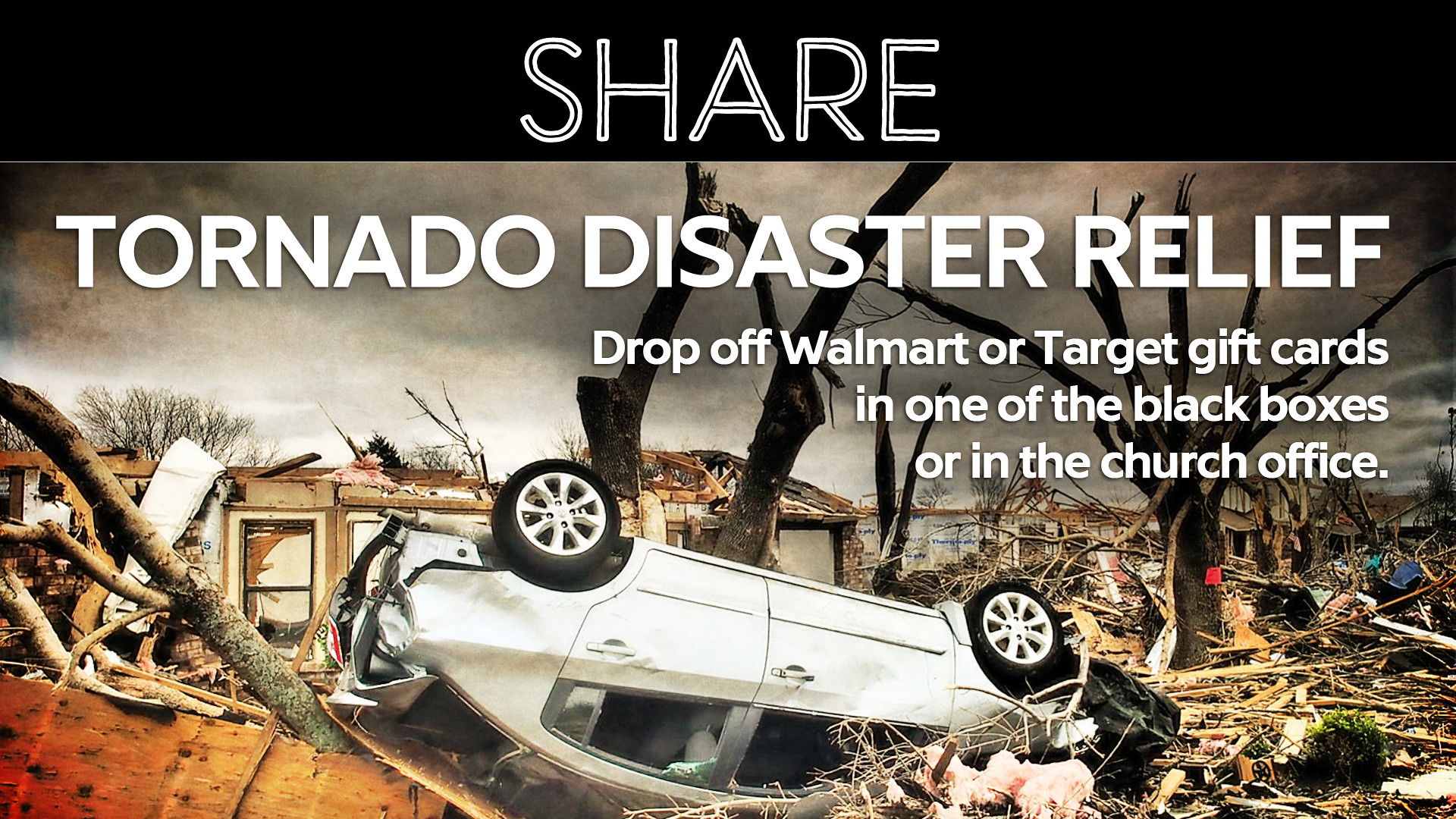This photograph, likely shared on social media for a fundraiser, captures the aftermath of a devastating tornado. In the center, an upside-down white sedan with its wheels in the air is prominently featured amidst a chaotic scene of destruction. Surrounding the car is extensive debris, including shattered wood, tree limbs, and remnants of personal belongings. The backdrop reveals what’s left of a house, almost entirely roofless and severely damaged. Trees in the area are stripped of branches and leaves, standing as stark reminders of the storm's power. The sky above is dark gray, adding to the somber mood. At the top of the image, a black banner with white text reads "SHARE," and over the chaotic scene, bold white text declares "TORNADO DISASTER RELIEF." In a smaller font beneath, it instructs viewers to "DROP OFF WALMART OR TARGET GIFT CARDS IN ONE OF THE BLACK BOXES OR IN THE CHURCH OFFICE." The combination of imagery and text underscores a strong appeal for aid in the face of this catastrophic event.